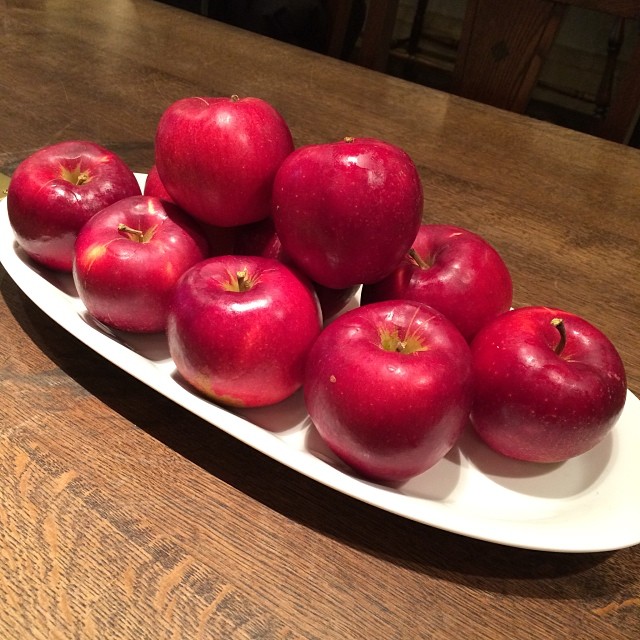Set against a well-lit dark brown oak table with visible grain patterns and light reflections, there's a long, oval white dish positioned horizontally. This dish is meticulously filled with ten bright red apples, arranged in a structured formation. The base layer consists of eight apples—arranged in two neat rows of four—topped with an additional two apples, making a pyramid-like stack. Some apples feature long, brown stems, while others are missing theirs, and one even has a slightly snapped stem. The apples exhibit a vibrant red hue, interspersed with occasional yellow and green spots where the skin is thin or scratched. The backdrop includes some seeding details on the table and a subtle, blurred hint of a chair on the top right, adding depth to the composition.